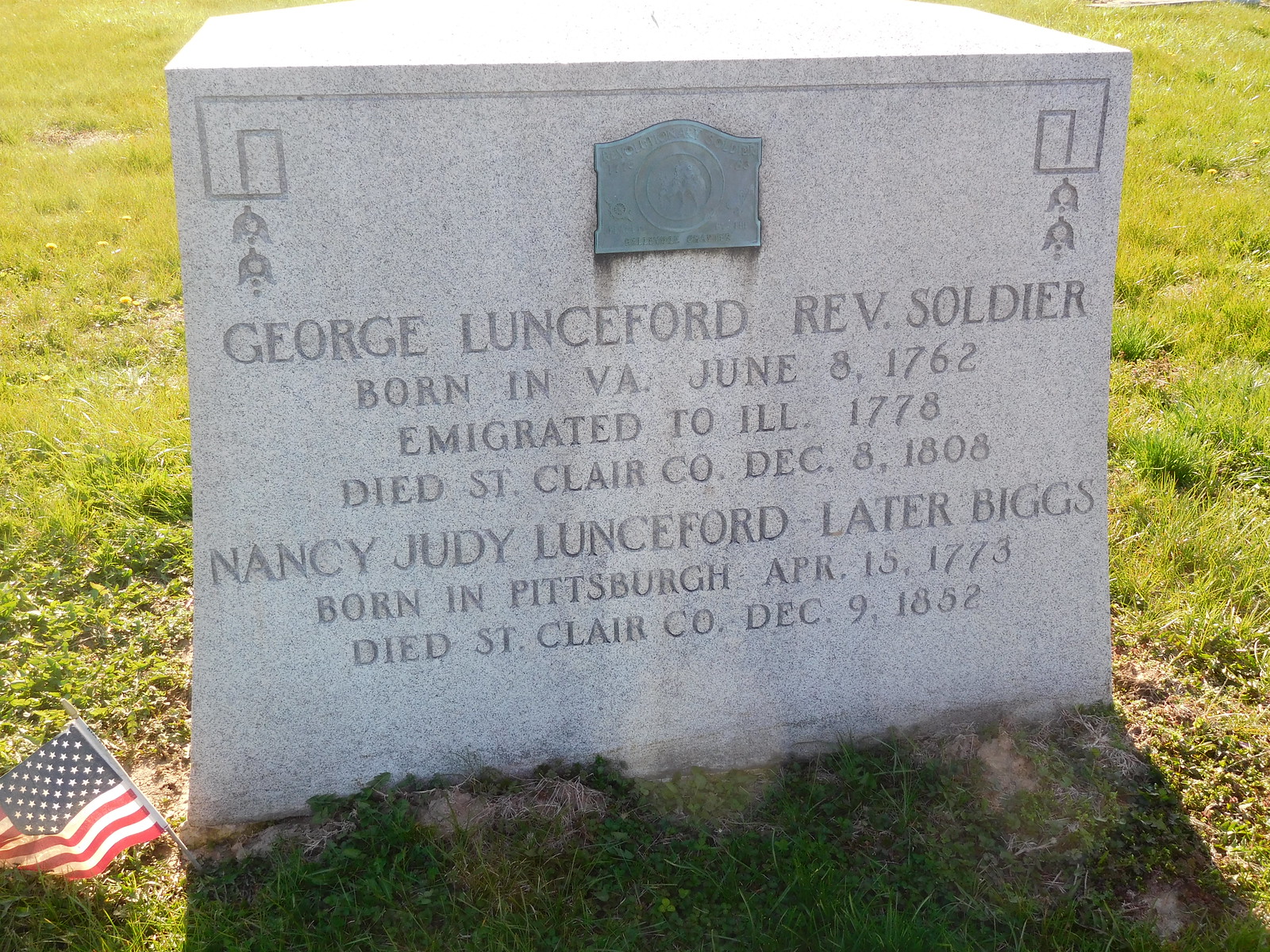This detailed headstone in a graveyard marks the final resting place of George Lunceford and Nancy Judy Lunceford, later Biggs. Surrounded by a lush expanse of green grass, it features an ornate vine design at the top and a blue plaque in the center. The light gray stone bears the inscription: "George Lunceford, Reverend Soldier, born in Virginia, June 8, 1762, emigrated to Illinois, 1778, died St. Clair, Colorado, December 8, 1808," and directly below is, "Nancy Judy Lunceford, later Biggs, born in Pittsburgh, April 15, 1773, died St. Clair, Colorado, December 9, 1852." A small American flag on a stick, placed at the bottom left corner of the stone, honors George’s service, completing the respectful and commemorative scene. Despite slight variations, the names and dates are consistently depicted across all captions.